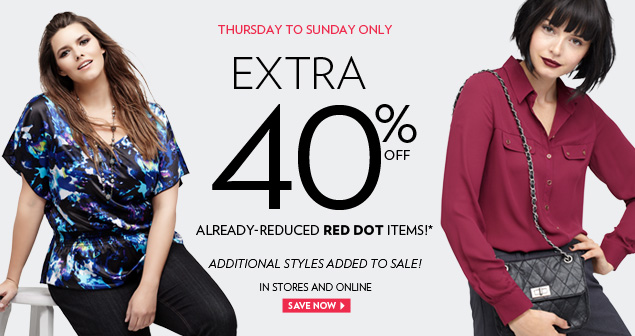This advertisement, set against a very pale gray background, features two striking models showcasing stylish apparel. On the left, a beautiful white woman with long, flowing hair pulled back from her face is dressed in a silky black, blue, and white short-sleeve top that is cinched at the waist. She pairs this with blue jeans and accessorizes with a delicate gold bracelet on her right arm, which rests against a white stool. On the right, another stunning white model with a pageboy haircut and bangs stands confidently. She has black hair, black eyebrows, and dark red lips, enhancing her dramatic look. She is wearing a burgundy button-up blouse, with the top two or three buttons stylishly undone, revealing placket pockets on her chest. Her ensemble is completed with dark charcoal dress pants and a quilted leather bag slung over her shoulder, the strap threaded through a silver chain. She accents her look with black fingernail polish, bringing a touch of edginess to her sophisticated outfit.